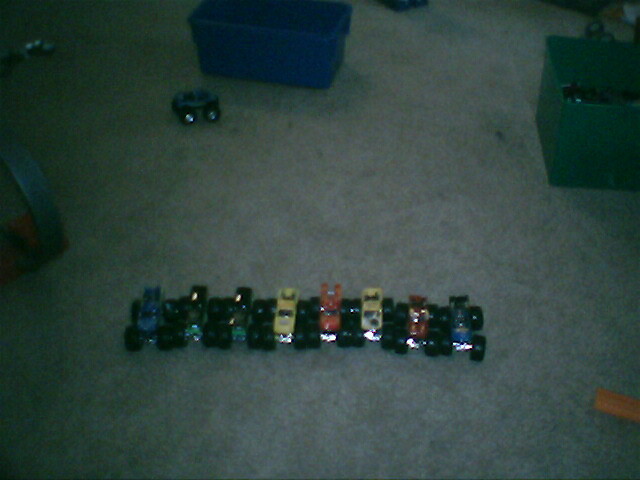In a slightly blurred photograph taken from above with a flash, you'll see a child's play area featuring a collection of vibrant toy monster trucks with oversized wheels. These trucks, in a variety of colors including blue, green, yellow, orange, red, and potentially black, are neatly lined up in a row towards the center-bottom of the image. One additional truck is positioned alone in the top left corner. The scene is set on a gray carpet, with a blue plastic bin and a green tote positioned near the center and top-right respectively, contributing to the playful and somewhat chaotic atmosphere. The image is devoid of any text.